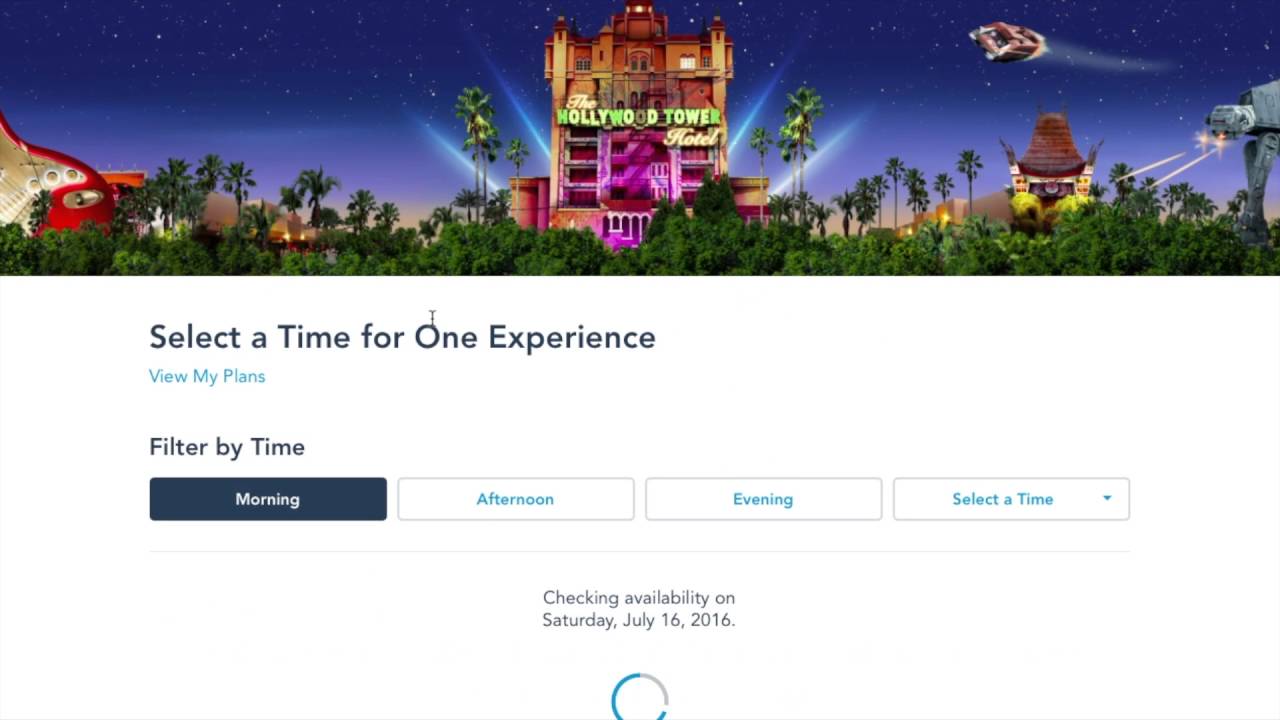The webpage features a vibrant image at the top, showcasing a Disney theme park. Dominating the scene is the iconic Hollywood Tower Hotel, a grand brown building illuminated with purple lights at the base. The landscape is lush with tall trees, including a number of palm trees. In contrast, a silver and red guitar stands prominently in the park, adding to the attraction.

The backdrop of the image is a deep blue sky adorned with twinkling stars, enhancing the magical atmosphere of the theme park.

Beneath the image is a user interface section, where visitors are prompted with "Select a time for one experience." A blue button labeled "View My Plans" is available for easy navigation. Additionally, a "Filter by Time" option allows users to choose from morning, afternoon, or evening slots via a dropdown menu.

Further down the page, the selected option is "morning," and the system is actively "Checking availability on Saturday, July 16, 2016." This is indicated by a half-filled circular loading icon, displaying a combination of blue and gray segments.

The primary design of the webpage features a clean, white background with blue text, creating a user-friendly experience. The topmost section is dominated by the colorful and enticing image of the theme park, highlighting the Hollywood Tower Hotel and myriad other attractions in vivid detail.